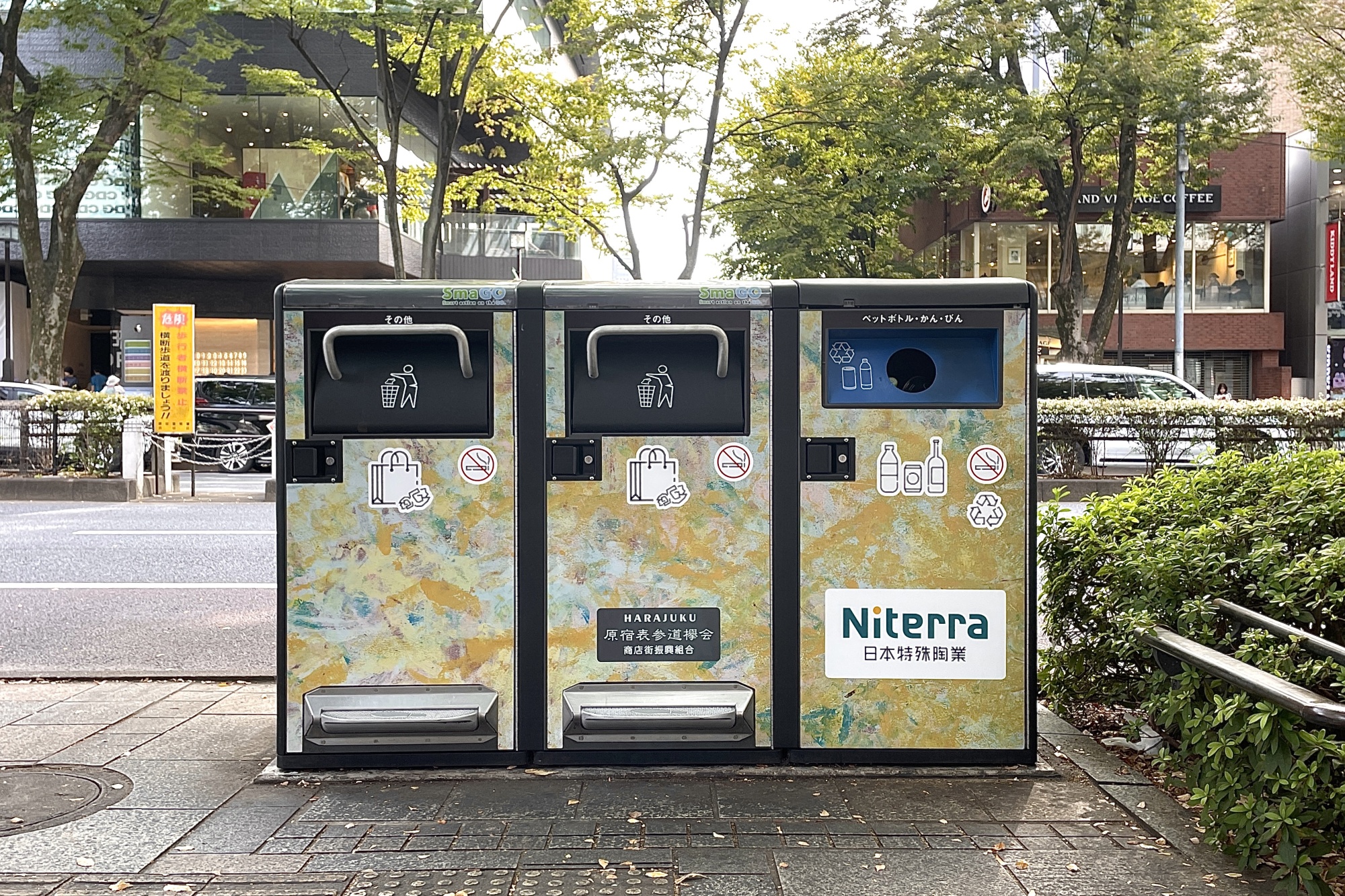This daytime photograph captures a set of three public trash and recycling bins positioned side by side on a gray sidewalk in an urban setting. The bins, labeled with the brand name "NITERRA," are composed of mixed colors: green, yellow, white, and metallic silver. The two bins on the left are designated for regular trash, featuring symbols indicating that lit smoking materials are prohibited. These bins have silver pull-down bars to access the trash compartment. The bin on the right is specifically for recyclables, marked with a blue recycling logo and additional text in Japanese or Chinese kanji.

In the background, the image shows a city street with a visible median, separating the photographed side from the opposite lane where a white car is driving. The street is framed by low-rise city buildings that showcase significant glass elements in their architecture, as well as various road signs in an East Asian script, likely Japanese or Chinese. A notable yellow road sign is positioned to the left side of the bins. Additionally, the scene is enriched with urban greenery, including several trees, creating a balanced portrayal of man-made and natural elements in a bustling city environment.